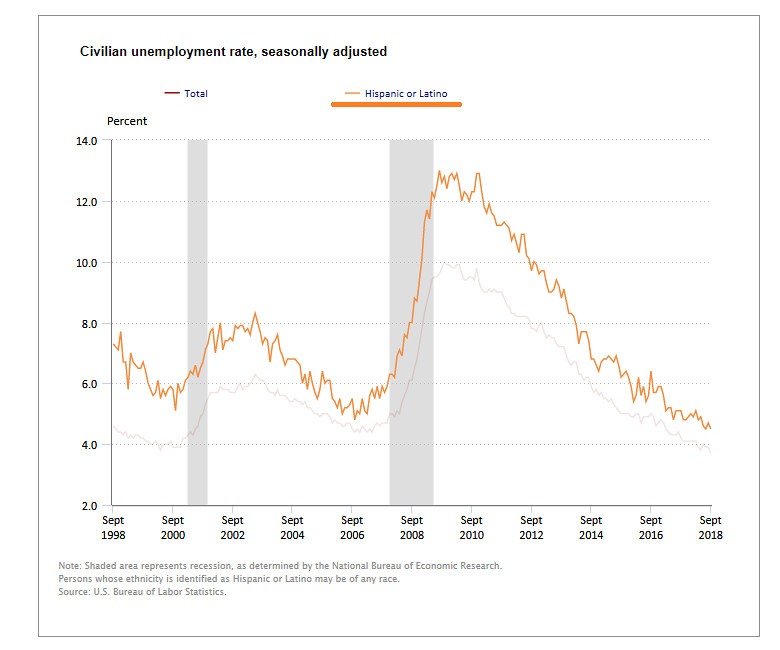The image is a detailed line graph titled "Civilian Unemployment Rate, Seasonally Adjusted," with data sourced from the U.S. Bureau of Labor Statistics. The graph features two lines: a dark orange line representing the total unemployment rate and an orange line for the Hispanic or Latino unemployment rate. The x-axis spans from September 1998 to September 2018, marked in two-year intervals, while the y-axis scales unemployment rates starting at 2.0%, increasing by increments of 2%, up to 14.0%.

Both lines start in September 1998 around the 6-7% range, with the Hispanic or Latino rate generally higher than the total rate throughout the period. The lines initially decline until September 2000, followed by a slight rise peaking in September 2002. They then dip to their lowest around September 2006 before sharply increasing to a peak in 2010, attributed to the aftermath of the economic recession. From that peak, the rates gradually decrease, continuing to fall until the endpoint in September 2018, where the total unemployment rate is around 4% and the Hispanic or Latino rate is approximately 5%.

Additionally, there is a shaded area marking recession periods as identified by the National Bureau of Economic Research. The graph also clarifies that individuals identified as Hispanic or Latino could belong to any race.